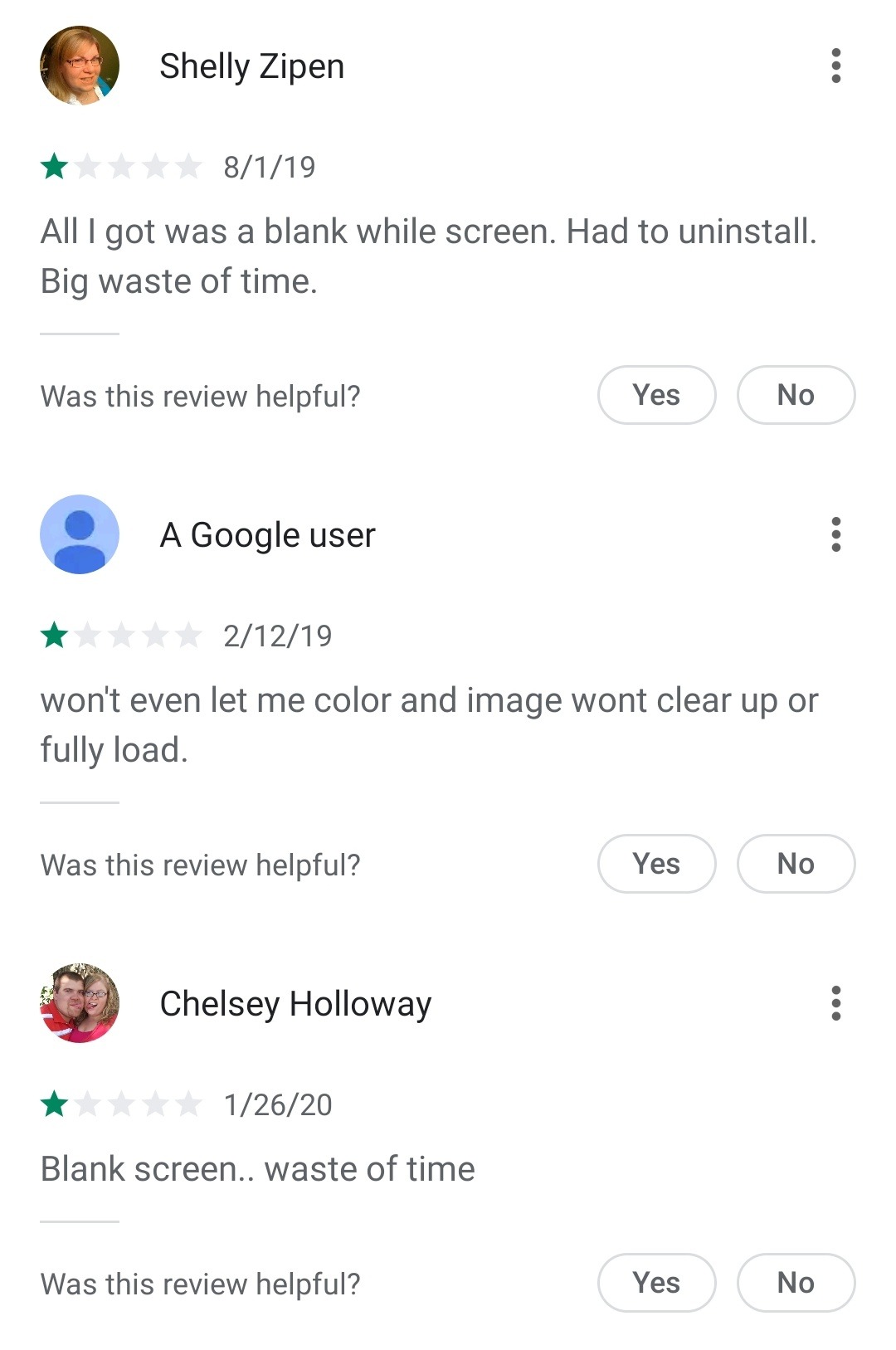This image showcases a column of three distinct user reviews for a product. Each review features a layout that includes the reviewer's avatar in a circular frame positioned on the upper left. To the right of the avatar is the reviewer's name, and further to the right are three vertically oriented dots which likely function to expand user information.

Below the name are five stars indicating the star rating, with the unselected stars in grey and the selected stars in green. The selected stars illustrate the rating given by each reviewer. Following the rating is the date of the review, and beneath that is the text of the review itself. A small horizontal grey line, taking up about 10% of the column width, separates the review from additional feedback options. Below this line, there is a query asking if the review was helpful, accompanied by two action buttons labeled "Yes" and "No" with a white fill.

The reviewers are Shelly Zippin, a Google user, and Chelsea Holloway, each leaving a one-star review. Shelly Zippin’s review, dated 8-1-19, shows a middle-aged female with glasses looking to the right. Her review states, "All I got was a blank screen. Had to uninstall, big waste of time."

The second review, dated 2-12-19, is from a generic "Google user," represented by the typical blue default Google avatar. This review reads, "Won't even let me color. An image won't clear up or fully load."

The last review, dated 1-26-20, is by Chelsea Holloway, whose image depicts a couple—a woman with glasses and a man with white facial hair, both wearing red shirts. Chelsea's review simply says, "Blank screen... waste of time."

Each of the three reviews highlights significant frustration, all lamenting a common issue of a blank or unresponsive screen, thus reflecting an overall negative user experience with the product.